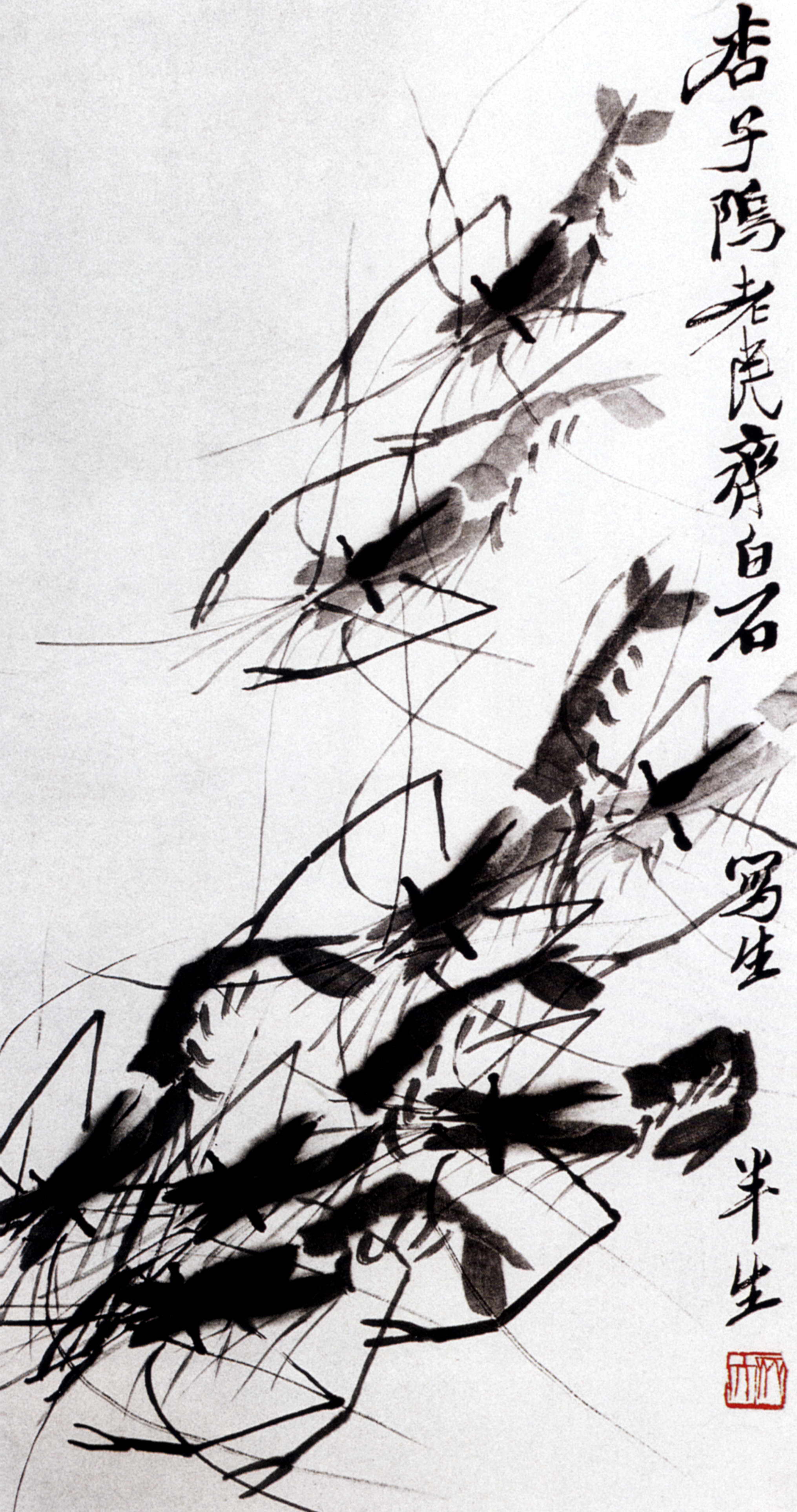An Asian ink painting featuring six shrimp dominates the composition, arranged diagonally from the top right to the bottom left. Executed in black ink against a background blending light tan and gray hues, the shrimp's detailed bodies, antennae, and tails evoke a delicate, x-ray-like quality. This artwork is accentuated by Asian text, which runs vertically along the right side from top to bottom, culminating in a prominent red character at the bottom right corner, adding a striking contrast to the monochromatic palette.